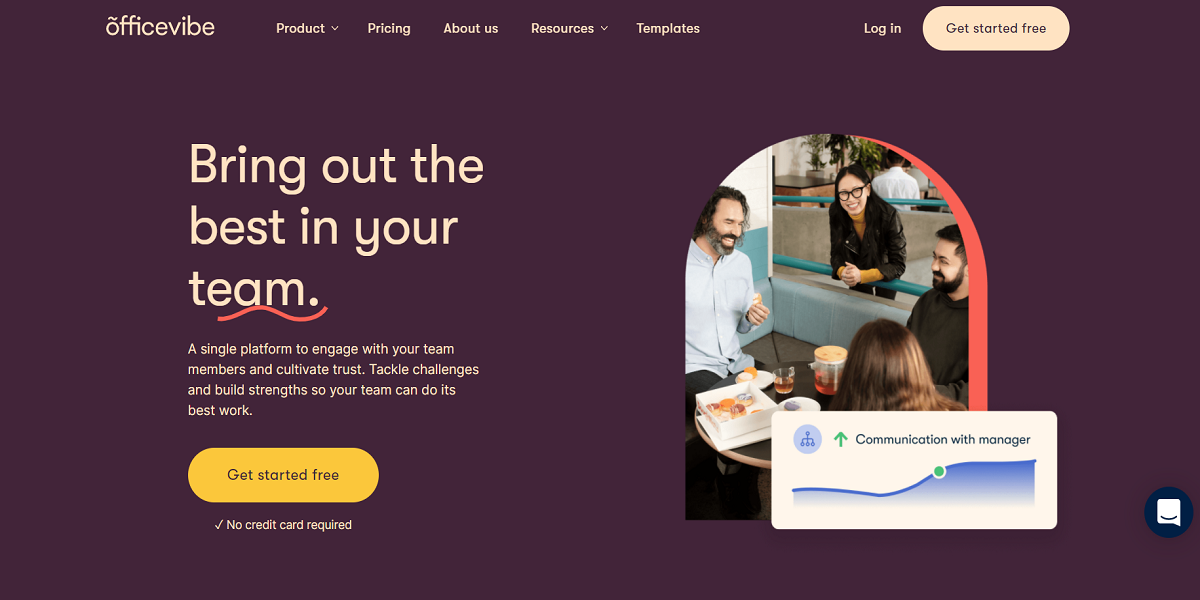The advertisement for Office Vibe features a maroon-themed background with taupe-colored text and elements. At the top, the words "Office Vibe" are prominently displayed, followed by navigation options: "Product," "Pricing," "About Us," "Resources," and "Templates." To the right, there are two call-to-action buttons – "Log In" and "Get Started for Free," the latter in taupe.

The main headline reads, "Bring Out the Best in Your Team," followed by a descriptive subtext: "A single platform to engage with your team members and cultivate trust. Tackle challenges and build strength so your team can do its best work. Get started free, and no credit card is required."

Below the text, an image depicts three people seated around a table with drinks, presumably tea. They appear to be in a discussion, and a thick book is placed on the table. Additionally, a woman is shown leaning over the rail adjacent to their table. Beneath the image, a box contains the caption "Communication with Manager" with an upward-pointing arrow, indicating improvement.

The overall design effectively emphasizes Office Vibe's focus on team engagement and communication.